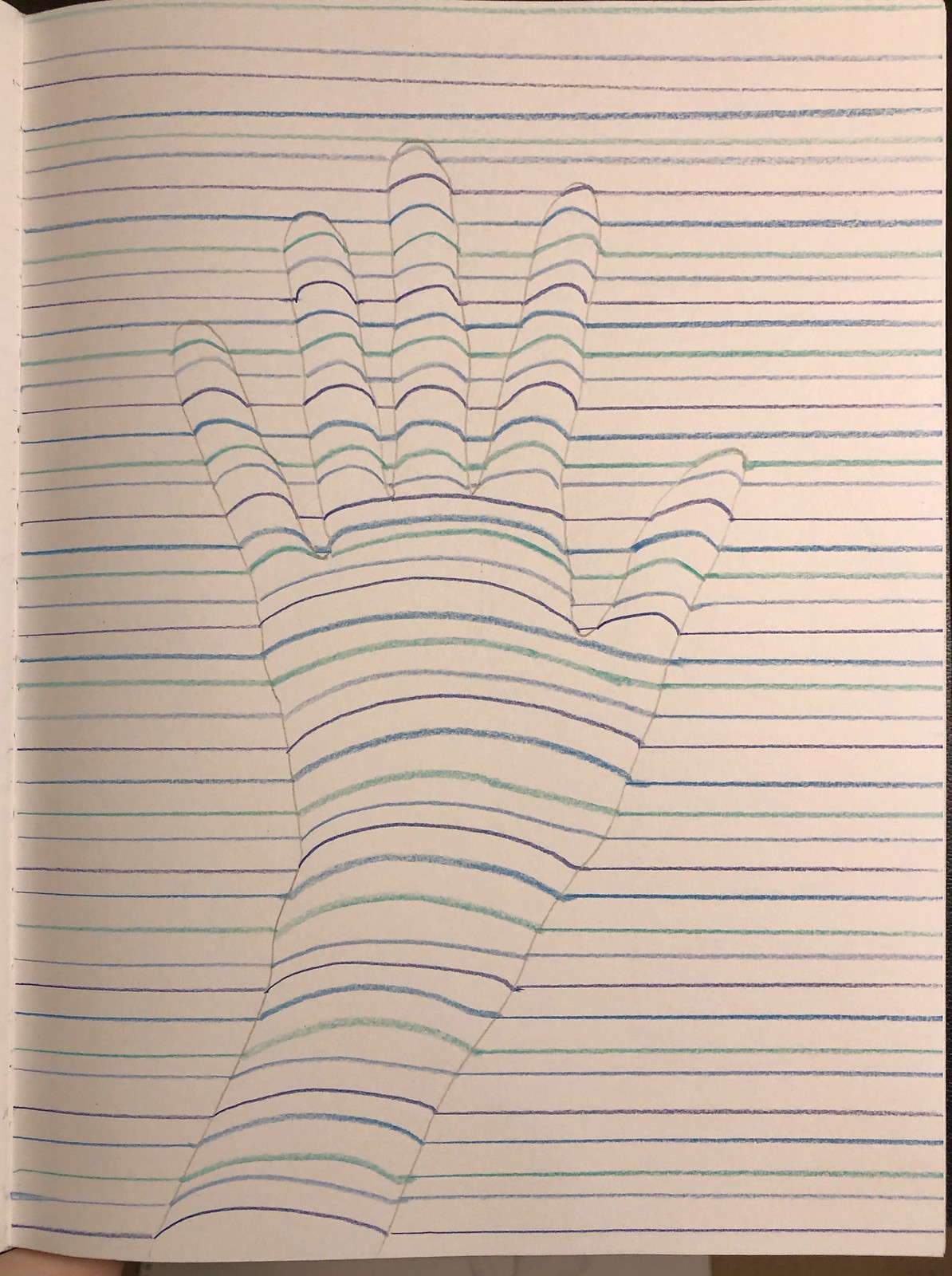A detailed and descriptive caption for the image:

"An intricate hand-drawn illustration of a human hand rendered on lined notebook paper, utilizing the contour line drawing technique. The lines on the notebook paper run horizontally, providing a structured background for the artwork. The hand is meticulously crafted using a series of curved parallel lines that create a compelling optical illusion, making the hand appear to rise from the flat surface of the page. These contour lines elegantly follow the natural contours and curves of the hand, fingers, and thumb, enhancing its three-dimensional effect. The drawing is executed in blue ink with delicate green highlights that trace the same contour pattern, adding a subtle variation in color and depth. This creative composition highlights the playful and artistic use of lines to suggest form and dimensionality."